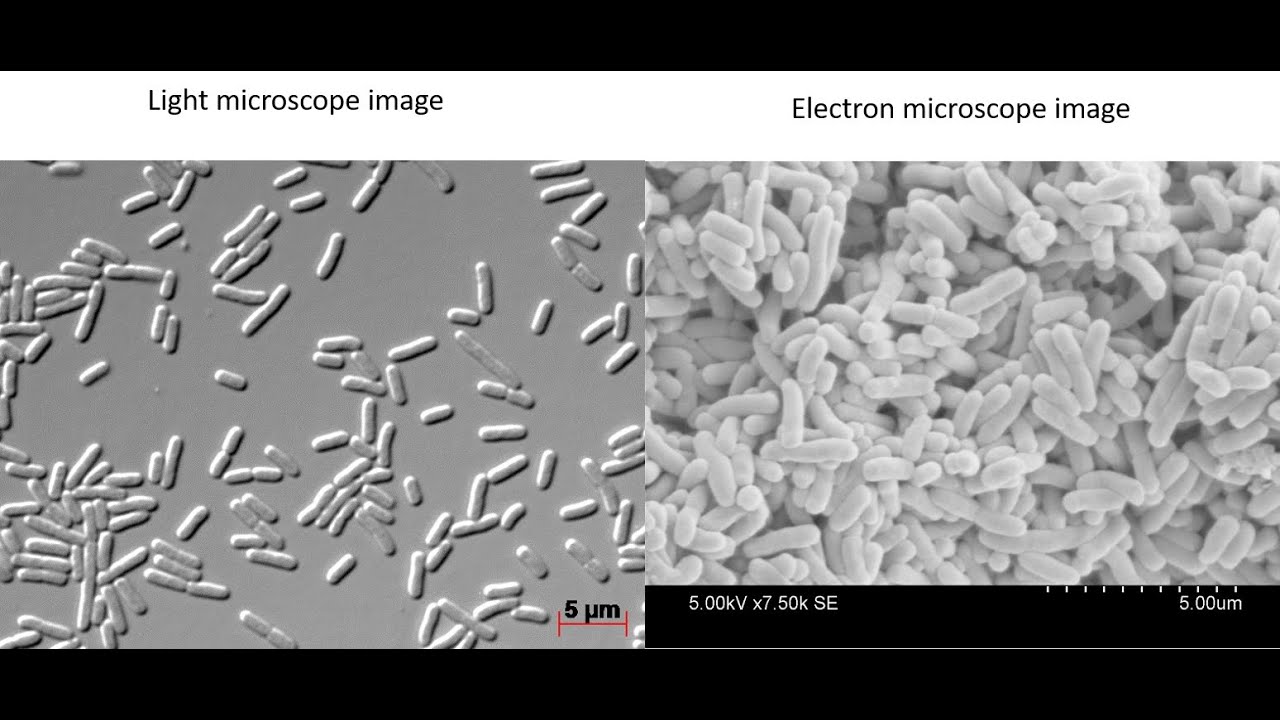This is a horizontally aligned rectangular image in black and white, designed to compare the details captured by a light microscope and an electron microscope. The image is bordered by thick black strips at the top and bottom. Directly below the top border, the left section is labeled "Light Microscope Image" while the right section is labeled "Electron Microscope Image."

Under each label, there are square photographs. The photograph on the left under the light microscope label features a dark gray background with white objects resembling elongated grains of rice or small capsules scattered throughout. In the lower right corner of this photograph, the scale is displayed as "5 micrometers" in bold text.

The photograph on the right under the electron microscope label offers a much closer, more detailed view. Here, the same cylindrical objects appear closely packed together, almost forming clusters, without a discernible background. The scale in the lower right corner of this photograph also reads "5.00 micrometers" and to the left of this, it states "5.00 kilovolts times 7.50 KSE." 

Overall, the electron microscope image provides far greater detail compared to the light microscope image, showcasing the texture and density of the cylindrical objects more clearly, akin to grains of rice closely packed together.